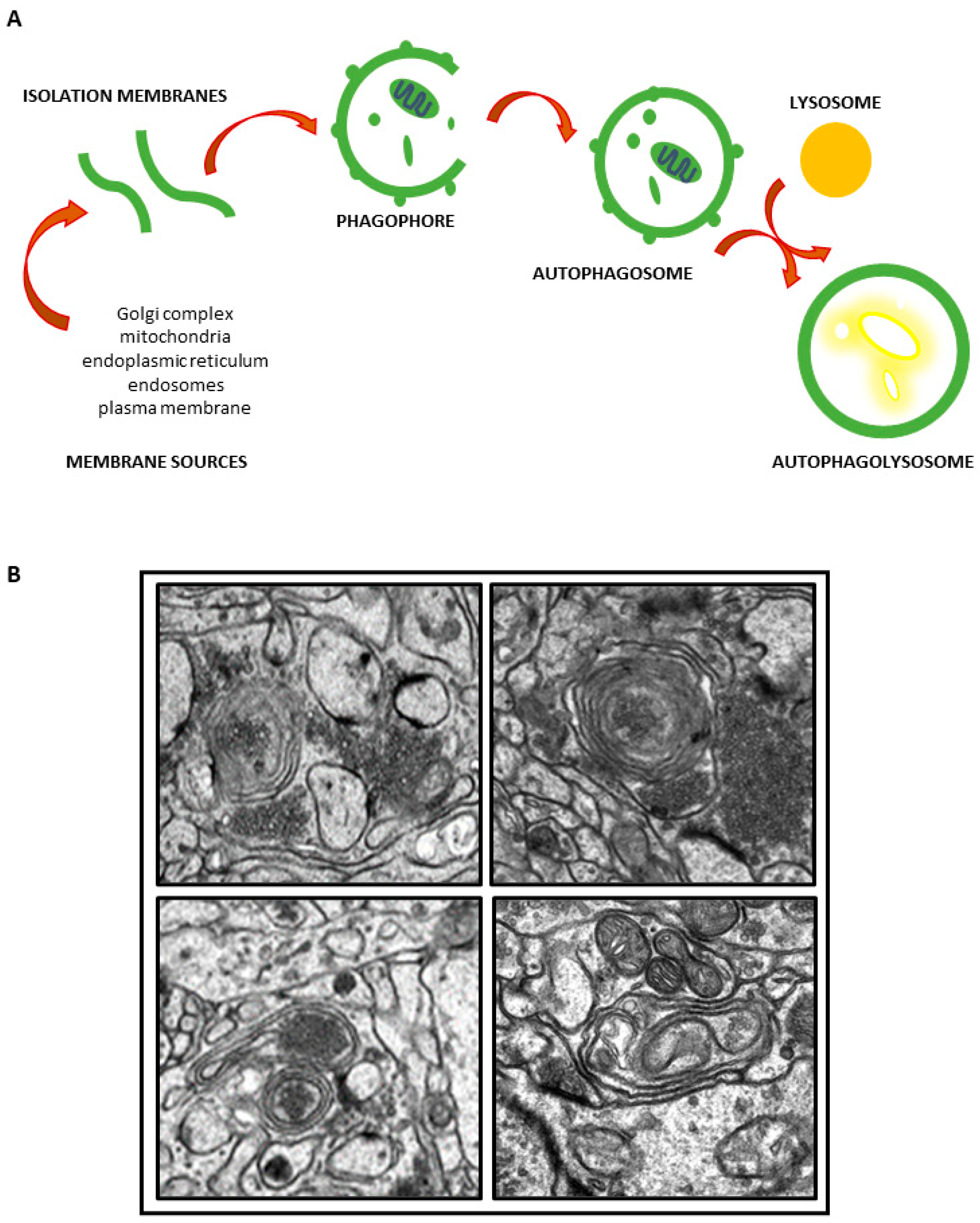The image features an intricate combination of multicolored text and black-and-white images, presented in a vertical rectangular format with a white background. The top section, labeled 'A', displays a detailed chart highlighting various cellular structures and processes, all under the general heading of "isolation membranes." This part of the image showcases several stages of cellular activity, including phagophore, autophagosome, autophagolysosome, and covers a range of cellular components such as the Golgi complex, mitochondria, endoplasmic reticulum, endosomes, and plasma membrane. The text is predominantly in black color, while the illustrations incorporate green lines, red arrows, and various other colored dots and shapes to highlight specific elements.

The bottom section, labeled 'B', consists of a grid of four square images, each separated by white lines. These are microscopic images that depict different types of cells, although the exact cell types are not specified. The images within these squares are in black and white with varying shades of grey, showing various cellular structures that appear in diverse shapes such as circles and ellipses. The entire composition is devoid of any external borders, relying on the background's white color to frame the content.